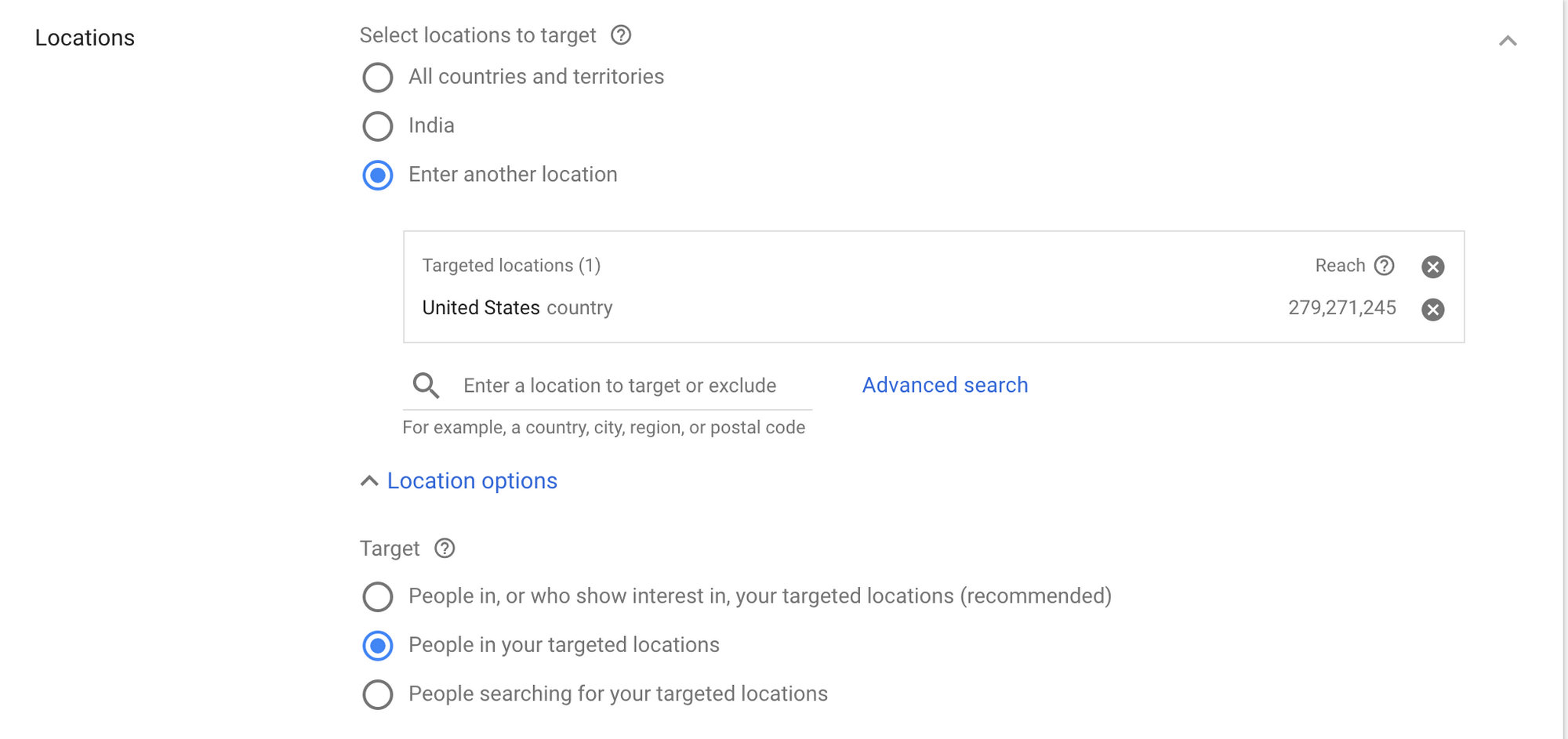This image displays a digital interface for setting advertising target locations. It showcases options to select and target specific locations, including countries and territories from a global list. The user has chosen India and the United States, with the United States showing a potential reach of 279,271,245 individuals. Additional options are available for inputting other locations or excluding certain areas. The platform targets individuals currently in the specified locations or those who have shown an interest in them. The recommended settings focus on people who are either in the targeted locations or searching for information about them.